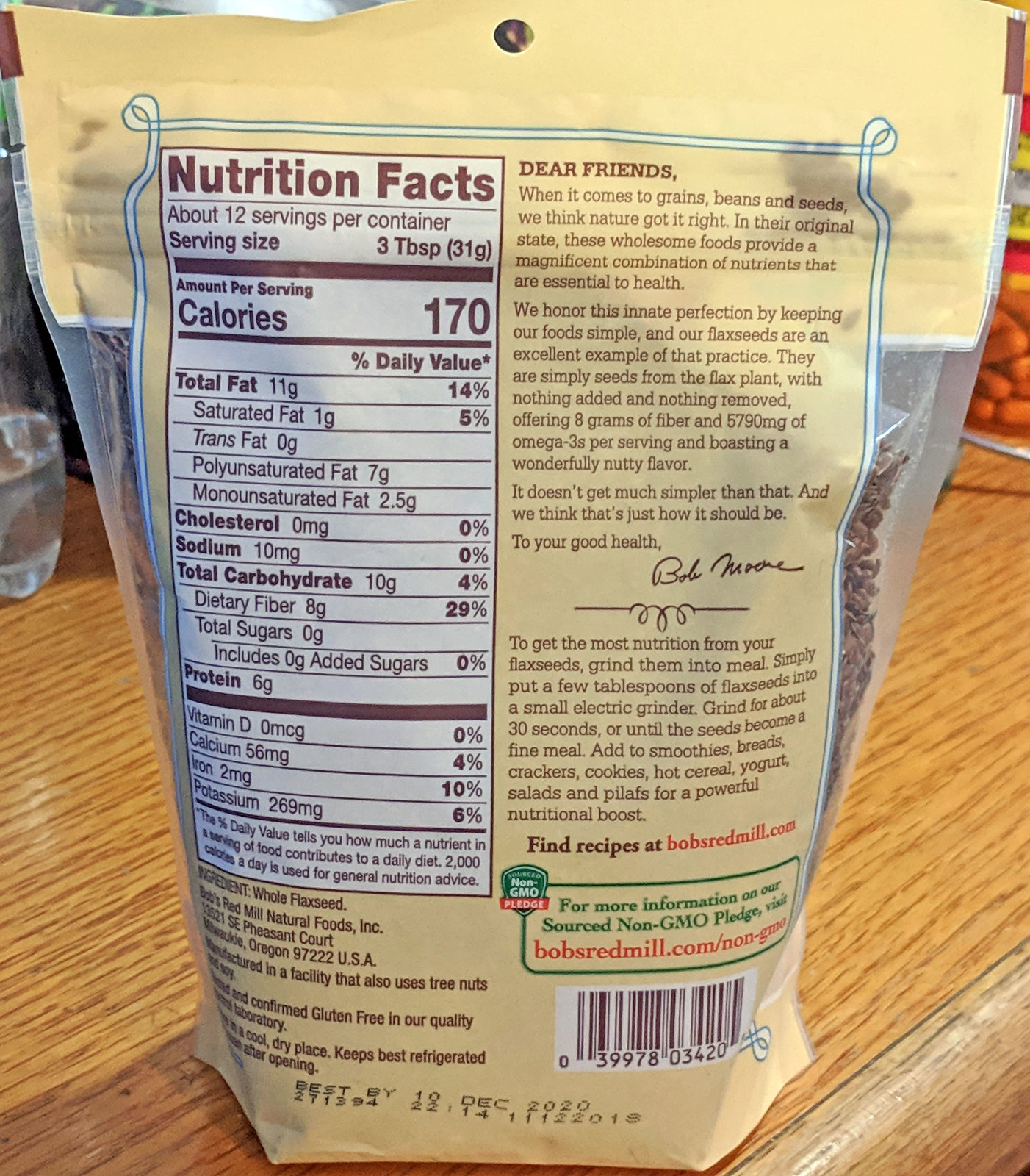This photograph features the back of a tan-colored pouch of flaxseed. On the left side of the pouch, there is a detailed table of nutritional facts printed in brown text on a white background. This table includes information on serving size, calories, total fat, cholesterol, sodium, carbohydrates, and protein content. On the right-hand side, there is a personal note from Bob Moore, the founder of Bob's Red Mill, which also mentions the website BobsRedMill.com for more information. The note pledges the product's non-GMO status and highlights its flavor and the wholesome nature of the food inside the package. At the bottom of the pouch, the "best by" date reads 10 December 2020. The pouch is resting on a wooden table, which is partially visible in the background.